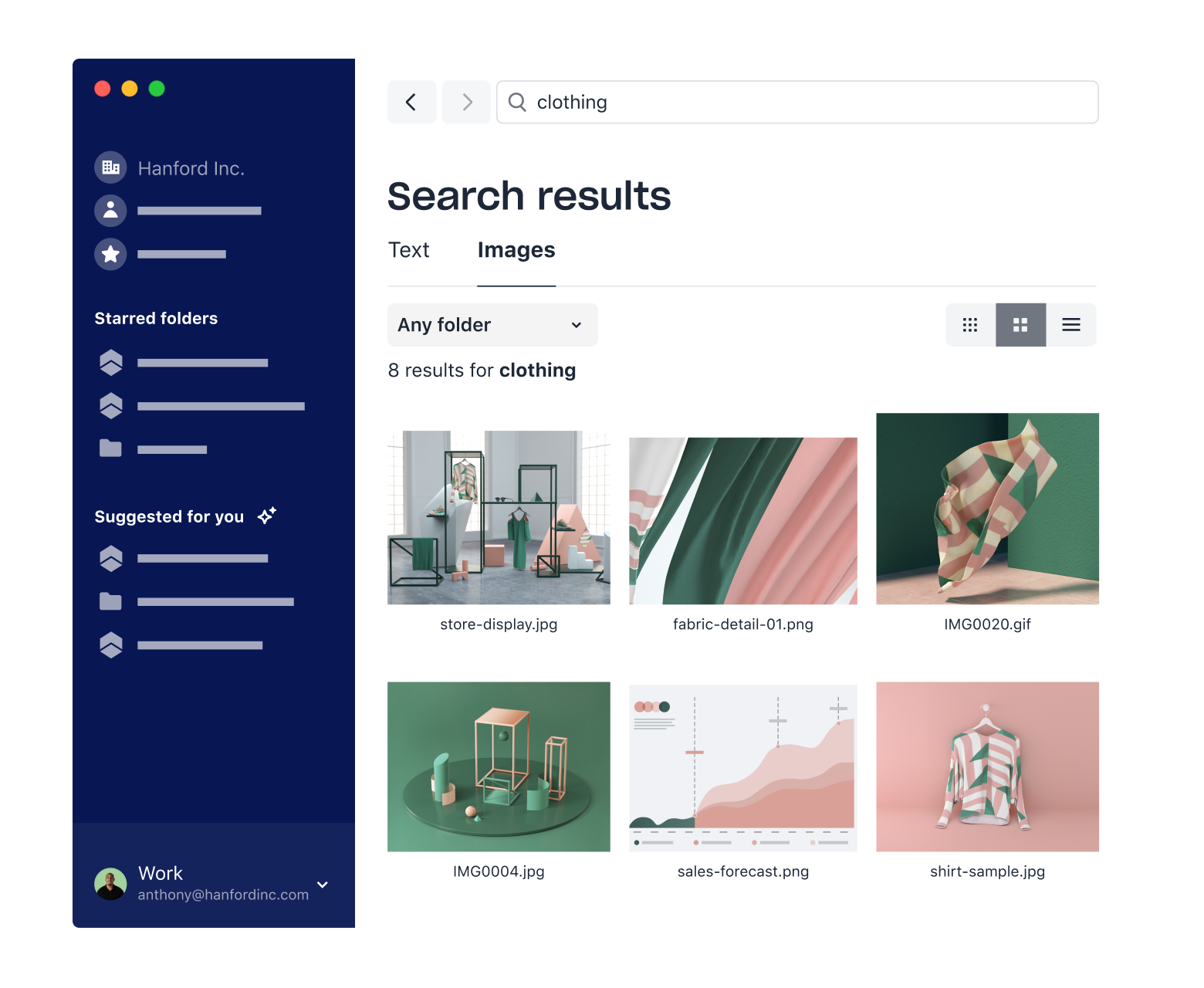This image is a detailed screenshot of a website interface. On the left side, there is a vertical blue sidebar that transitions from a navy blue at the top to a slightly lighter shade of blue at the bottom. At the very bottom of the sidebar, the word "Work" is displayed in white text next to the user's email address. A small photo of a man, possibly a white male, wearing a blue-black shirt is featured here.

At the top of the sidebar, there are three dots in a vertical row, colored red, yellow, and green, respectively. Below these dots, the company's name, "Hand Poured Ink," is written in a light blue font. Underneath the company name, several icons are visible, including one for "Account." A headline in white font reads "Shared Folders," followed by another section labeled "Suggested for You" further down.

The main content area takes up about three-quarters of the page, with a predominantly white background. The search results section is displayed here, indicating that the term "clothing" was used. The header says "8 results for clothing" in gray font. The page is currently on the "Images" view, as opposed to the "Text" view.

Six images appear in the search results, and they are somewhat abstract in nature. The first image shows a store display, which appears to be more of a simple drawing than a photograph. The second image is labeled "Fabric Detail" and is also a drawing. Another result, "Sales Forecast," features a graph with shades of blue, pink, and gray. Lastly, the bottom right image is titled "Shirt Sample," depicting a shirt in tones of pink, white, and gray, which seems to be a drawing as well.